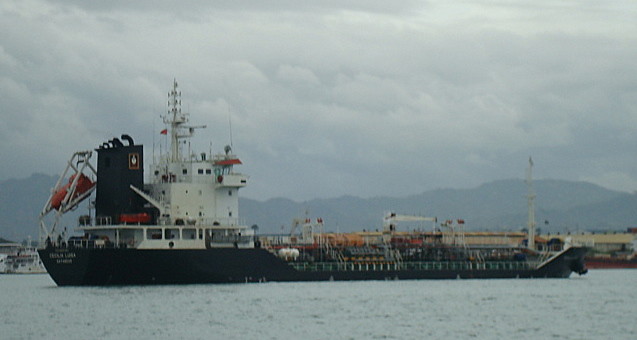This image is a horizontally aligned rectangular photograph capturing a large cargo ship navigating choppy waters under an overcast sky. The foreground features the ship with a black bottom section and a white upper section, including some tall white rectangles and a flat back end. Despite the distance, there is some unreadable white writing on the front of the ship. Additionally, a lifeboat is mounted at the rear of the vessel, poised for emergency deployment. The turbulent water surrounding the ship is visibly unsettled, with waves cresting at the bottom of the image. The sky above is thick with puffy gray and white clouds, contributing to the overall grayish tone of the picture. In the background, the hazy outline of distant hills can be seen, adding depth to the scene.